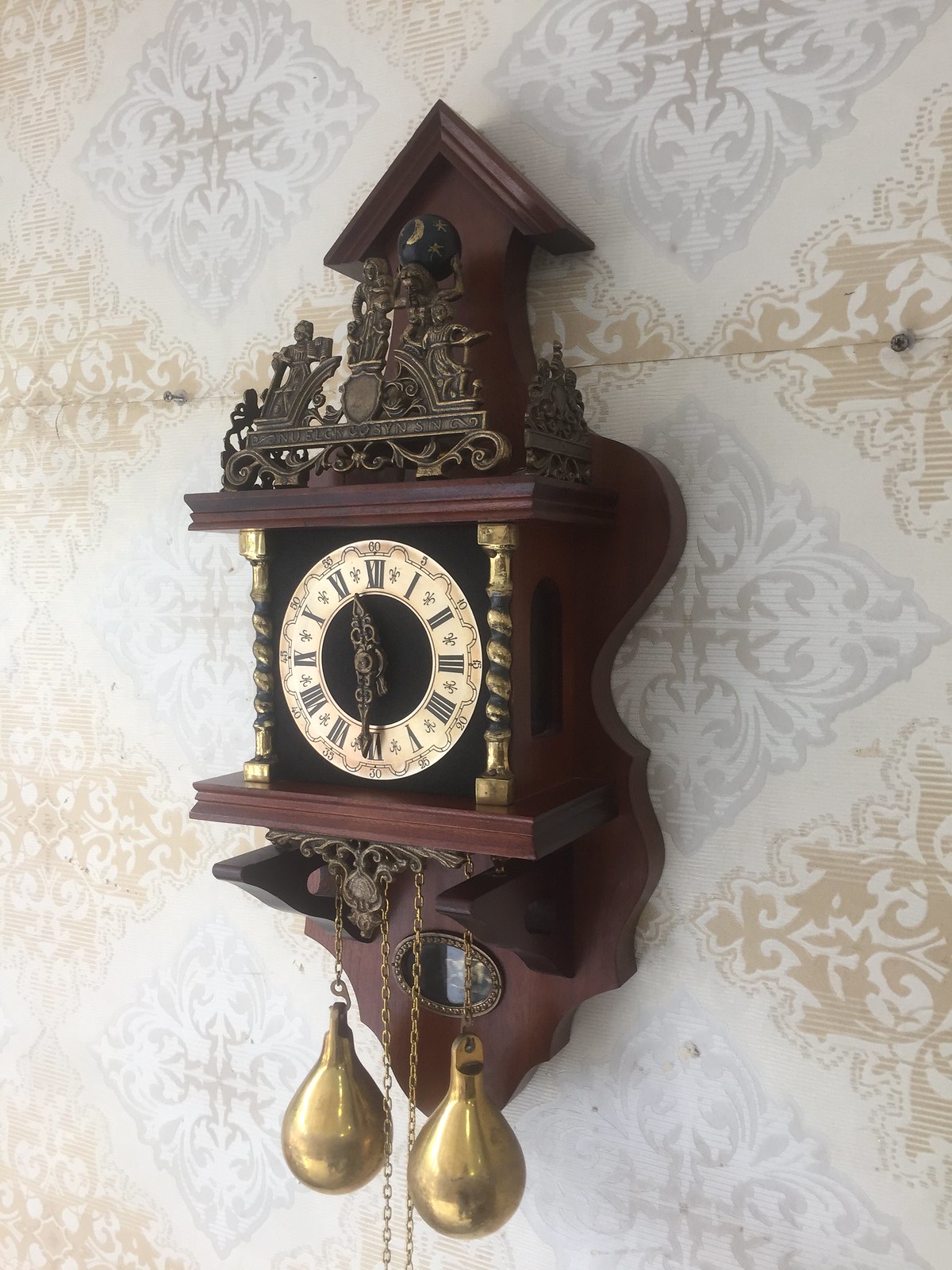Centrally positioned in the vertical, rectangular photograph is a beautifully intricate cuckoo clock, suspended on a wall adorned with white wallpaper featuring alternating silver and brown diamond designs. The clock's top, reminiscent of a house's roof, slopes gracefully into its square sides and highly sophisticated face, which showcases ornate Roman numerals indicating 11:30. Below the clock face, the structure tapers into an upside-down triangle, culminating in two elegantly dangling weights and a chain. The delicate craftsmanship merges with the nuanced details of the wallpaper background, creating a harmonious and visually striking composition.